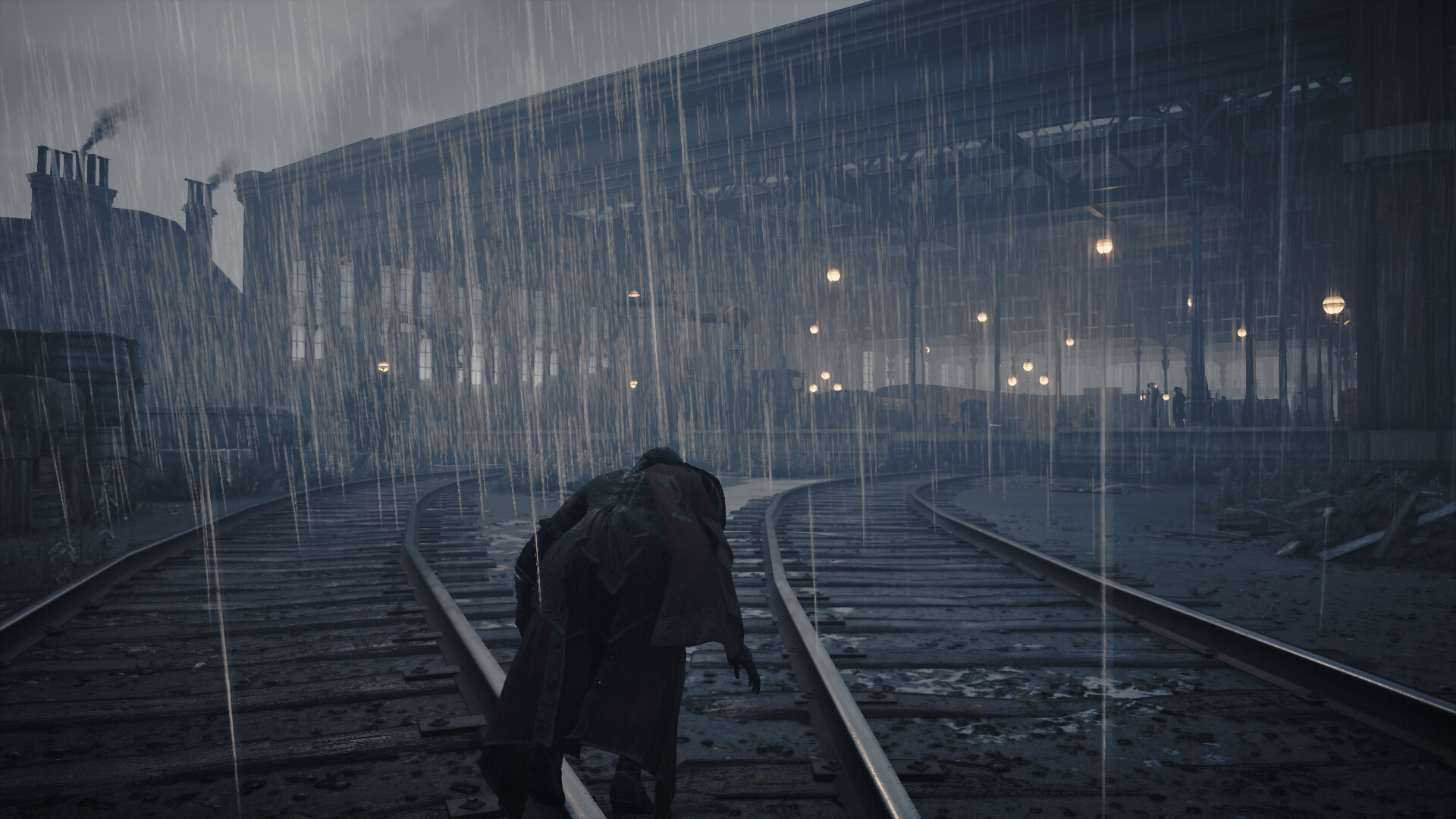In this meticulously detailed digital artwork, a solitary figure is depicted walking through a rain-soaked train depot under an ominous sky, suffused with shades of blue and grey. The person, appearing forlorn and somewhat odd, is hunched over, trudging towards the station without an umbrella, likely drenched from the torrential downpour. The setting seems both timeless and eerie, with the depot highlighted by dim, yellow lantern lights that cast a muted glow against the night or the gloomy day sky.

In the near distance, the train depot features a partially open roof, allowing rain to fall ominously within. Adjacent to this, a set of structures with thatched roofs and numerous old-fashioned chimneys spew forth wisps of smoke, adding to the scene's vintage and somewhat ghostly ambiance. The combination of the forlorn figure, the relentless rain, and the melancholic palette creates a deeply atmospheric and haunting tableau, devoid of any text or additional context, leaving much to the viewer's imagination.